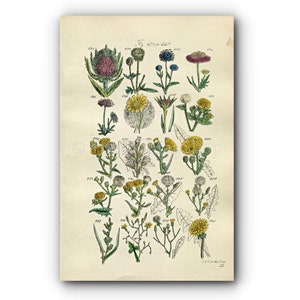The image shows an artist's rendering, possibly from a vintage guidebook or poster, featuring 20 different types of lush and blooming flowers arranged neatly in a 5x4 grid. Set against a paper-white to tan background, each floral illustration is meticulously detailed with vibrant colors, including hues of yellow, pink, white, blue, deep rose, and green. Despite the labels being illegible, the diversity and beauty of each flower are evident. Among them are recognizable flowers resembling sunflowers and daffodils, as well as unique varieties like a particularly striking flower that is green around the base, vibrant purple in the middle, and again green on the top. Each flower is accompanied by green foliage, adding to the lush appearance. The overall presentation of the flowers, all in full bloom, evokes the feel of a classic botanical guide.